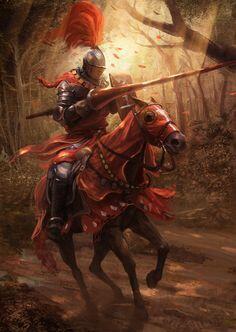Here we have a detailed artistic rendition of a knight in gleaming silver armor mounted on a horse, poised as if ready to joust with his lance extending forward. The knight is distinguished by a vibrant red plume of hair emanating from the top of his helmet and a matching red cape draped over his shoulders. The horse mirrors this color scheme, adorned with a red hood that covers its face save for openings for its eyes and a flowing red cloak extending down its head and body.

The scene is set in a dense, brown-hued forest, where light filters through the heavy canopy in striking god rays, casting a warm yellow glow onto the surroundings. The ground beneath the horse's hooves appears to be composed of a brownish-red dirt, resembling clay. This combination of natural and dramatic lighting enhances the vividness of the knight's red attire and the overall tension of the moment. The image, whether a painting or a digitally generated artwork, captures not just the knight and his steed but also the dynamic atmosphere of their woodland path.